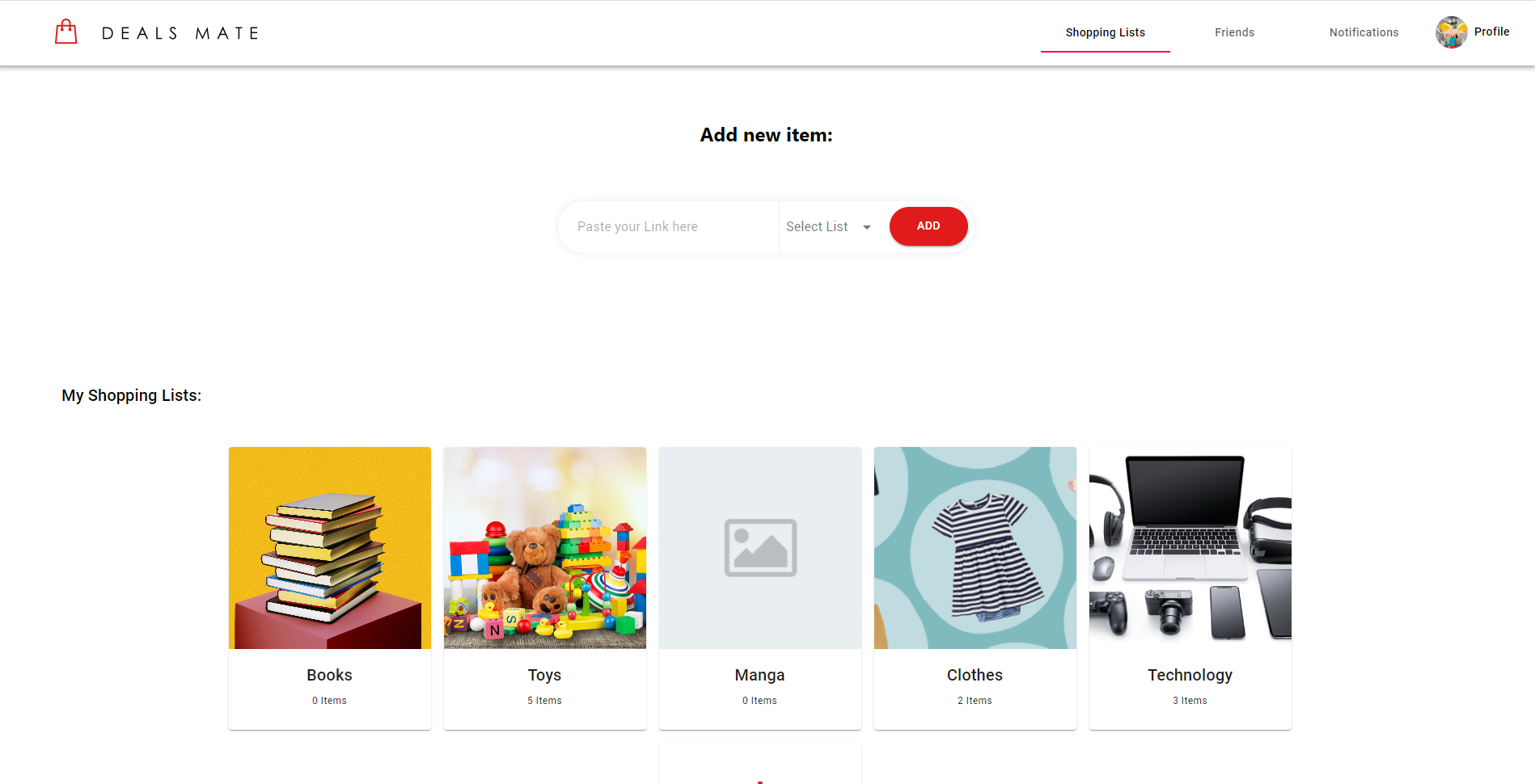The screenshot from DealsMate, a shopping website, features several navigation tabs at the top, including Shopping Lists, Friends, Notifications, and Profile. Below these tabs is a section to add new items, where users can paste links. The shopping list is organized into self-created categories, each represented with an icon and an illustrative image. 

The categories displayed include:
- **Books:** Represented by an image of a pile of books set against a yellow background on a red cube.
- **Toys:** Depicted with teddy bears, Lego blocks, and other toddler toys.
- **Manga:** (Image not specified in detail).
- **Clothes:** (Image not specified in detail).
- **Technology:** Featured with a laptop, camera, and other gadgets.

Each category shows the number of items saved, with Clothes having 2 items, Technology 3 items, and Toys 5 items.